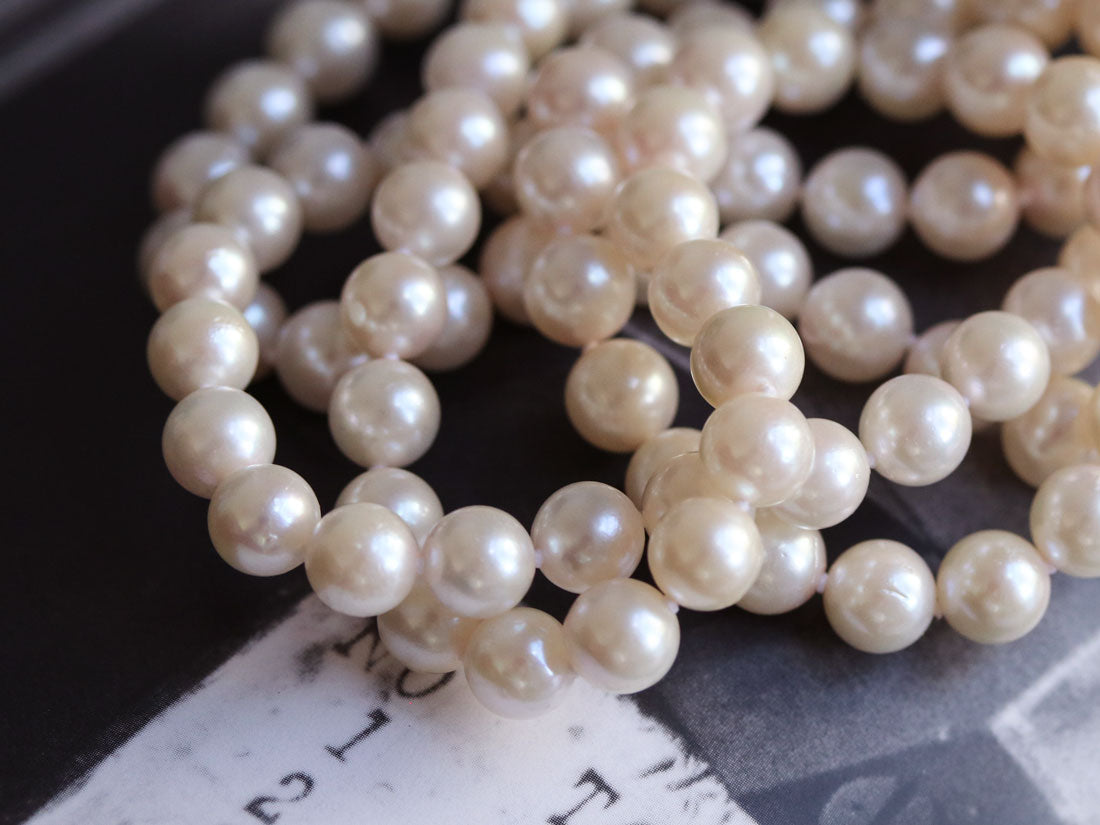The image is a detailed, close-up photograph of a collection of pearl necklaces draped over a dark gray base or table that takes up the majority of the scene. The pearls, cream-colored with a slightly yellow hue indicative of their age, are piled from the upper right corner of the image towards the bottom left, resembling a tangled heap. The pearls exhibit a noticeable shine and are most detailed and focused towards the center of the image. In the lower left corner, there's a piece of paper resembling an old-timey, stamped receipt marked with the letters "N-O," the numbers "1" and "2," and the letter "T," though the rest of the information is cut off. The background consists of the aforementioned gray surface, which might be leather, providing a vintage, ruddy aesthetic to the composition. The photograph appears to be taken in natural daylight, adding to the clarity and detail of the pearls.